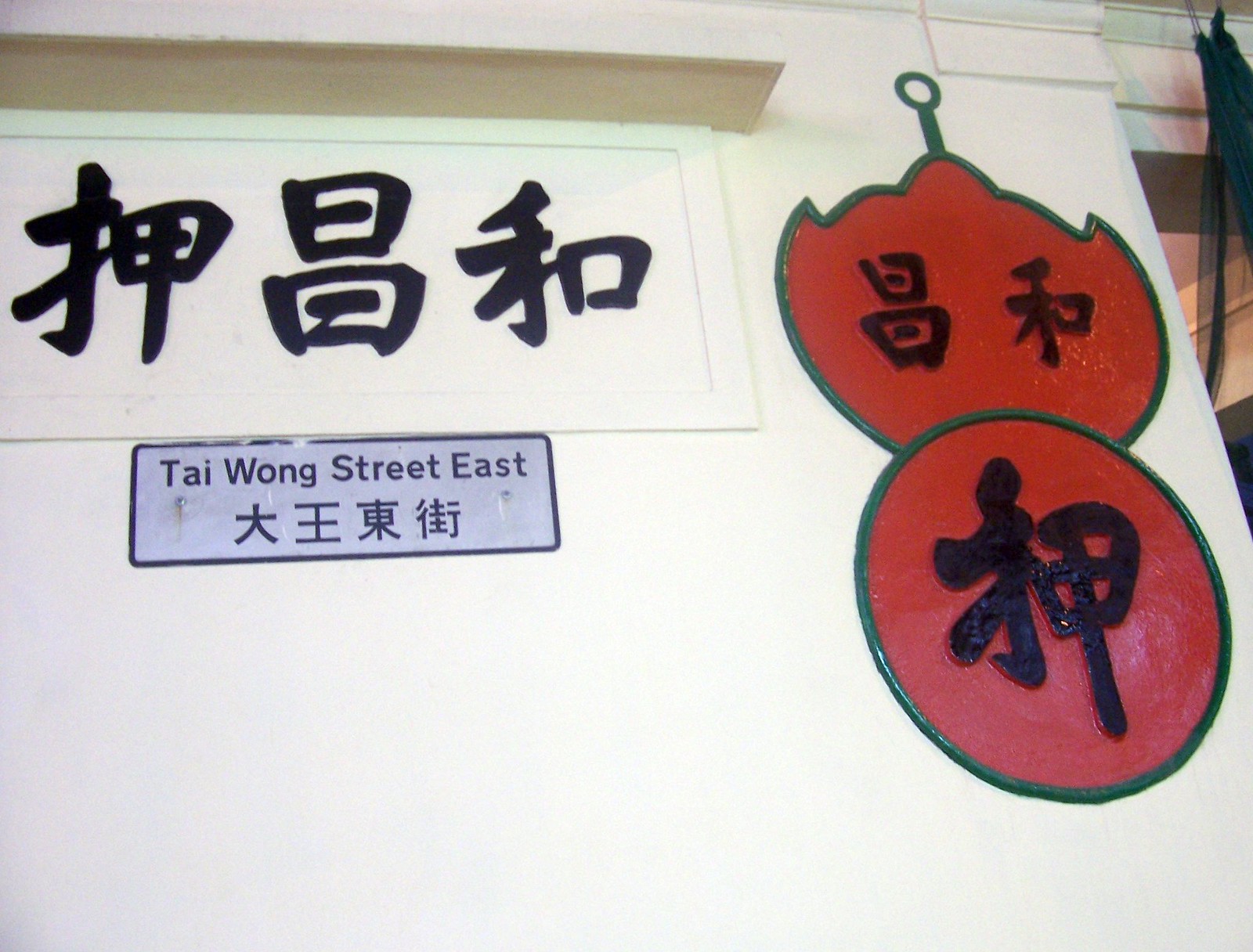The photograph depicts the facade of an outdoor building in China, featuring striking Asian iconography on a pristine white wall. On the left side of the image, three large Chinese characters are prominently displayed in black. Beneath these characters, a gray metal street sign bordered in black reads "Taiwan Street East" in English, with additional Chinese writing below it. To the right, the wall showcases what appears to be a part of an artistic installation: a red circle with a green border containing Chinese symbols, and above this, a green-handled semicircle with similar iconography. The vivid red and green elements, alongside the compelling black Chinese characters, contrast sharply against the bright, clean white facade, creating a visually captivating scene.